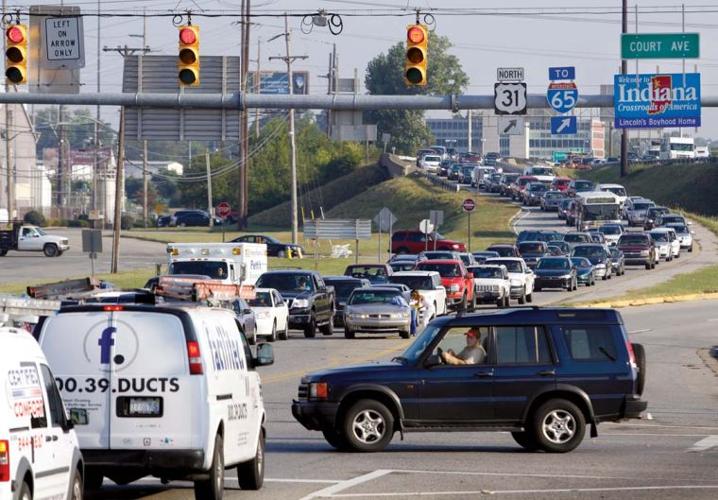This is a photo capturing a congested intersection in Indiana, possibly near the state line as suggested by a "Welcome to Indiana" sign. The traffic is heavily backed up, with vehicles halted at a red light, indicated by multiple stoplights overhead. Prominent signs include "Court Avenue," a directional sign for North Route 31, and an interstate sign pointing to Interstate 65, both exits leading off to the right.

In the scene, a black SUV in the foreground appears to be attempting a left turn, while an identifiable white panel truck, with partial text "00.39.ducts" and a logo, is also in sight. There is speculated oncoming traffic, potentially including an ambulance waiting at the light. 

The background features a cityscape with middle to tall buildings, emphasizing not skyscrapers but a more urban environment. Additionally, a sign indicating "Left on arrow only" provides driving instructions. The overall image reflects significant traffic congestion, indicative of peak travel times such as early morning or late afternoon.